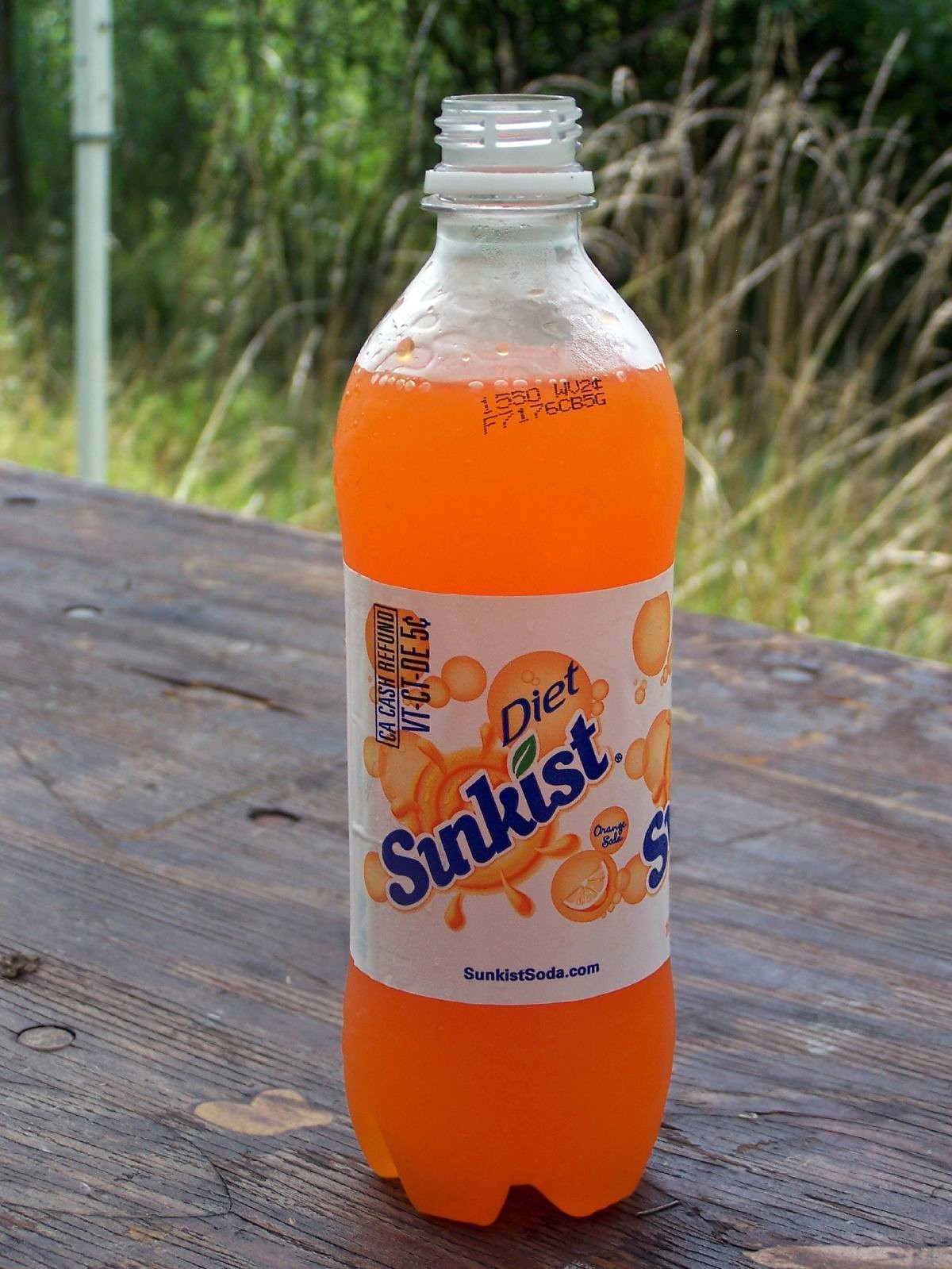The photograph, taken outdoors during the day, features a recently opened bottle of Diet Sunkist Orange Soda. The soda is housed in a tall, clear plastic bottle that lacks a cap, indicating it was just opened. The bottle is adorned with a white label in the middle, decorated with small orange bubbles and the branding "Diet Sunkist." Prominently displayed on the label are the words "California Cash Refund 5¢" and the website "sunkistsoda.com." Near the top of the bottle, there is a code reading "1550 WV 2 cents F717 6CB5G." The bottle rests on a wooden table, and the background showcases an expanse of tall grass, adding a natural element to the scene.